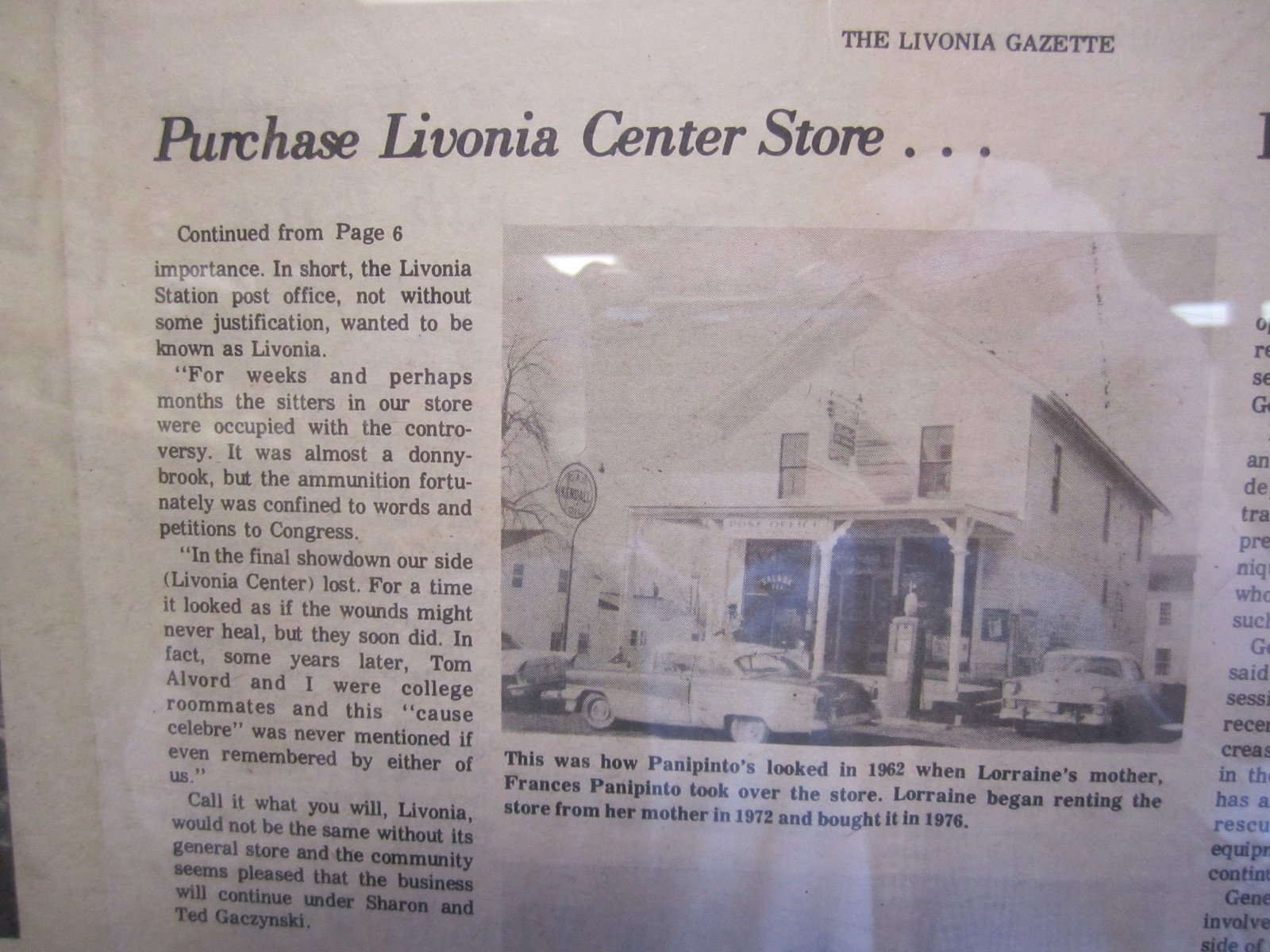The image is a framed newspaper article from the Livonia Gazette, showcasing historical details about the Livonia Center Store. The article, labeled "Purchase Livonia Center Store," suggests it has continued from page six and features multiple paragraphs of black text. A headline at the top right adds prominence to the story. A notable black-and-white photograph is included, depicting the Panepinto's store as it looked in 1962 with several cars parked outside, a gas pump in front, and a street sign nearby. The caption beneath the photo explains that Lorraine's mother, Frances Panepinto, took over the store in 1962. Lorraine then rented the store from her mother starting in 1972 and bought it in 1976. The presence of a reflective surface hints that the article is framed. To the right of the photograph, there are additional text columns that extend off the visible portion of the image.